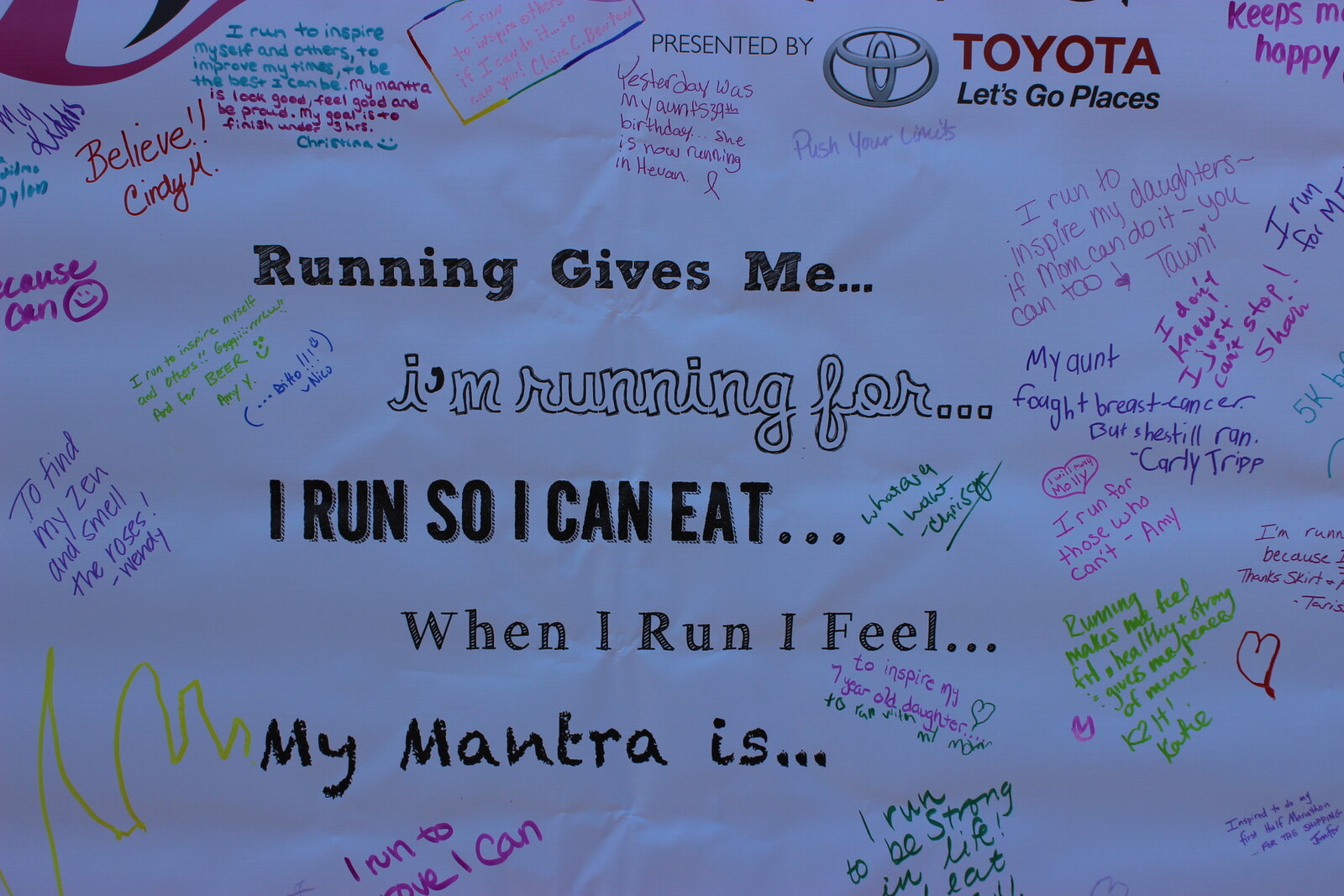The image showcases a banner, prominently displayed in what appears to be a Toyota dealership, as evidenced by the "Toyota, Let's Go Places" logo on the top right corner along with the text "Presented by Toyota." This banner is part of a charity event, likely a marathon aimed at raising money, possibly for breast cancer awareness, given the personalized and motivational messages related to health and strength. The banner has five mantra prompts printed in bold text: "Running gives me," "I'm running for," "I run so I can eat," "When I run I feel," and "My mantra is." Numerous individuals have signed the banner, completing these prompts with personal motivations and messages such as "I run to inspire my daughters," "My aunt fought breast cancer, but she still ran," and "Believe." These handwritten notes, although some are small and not easily decipherable, collectively create an inspiring collage of support and determination.